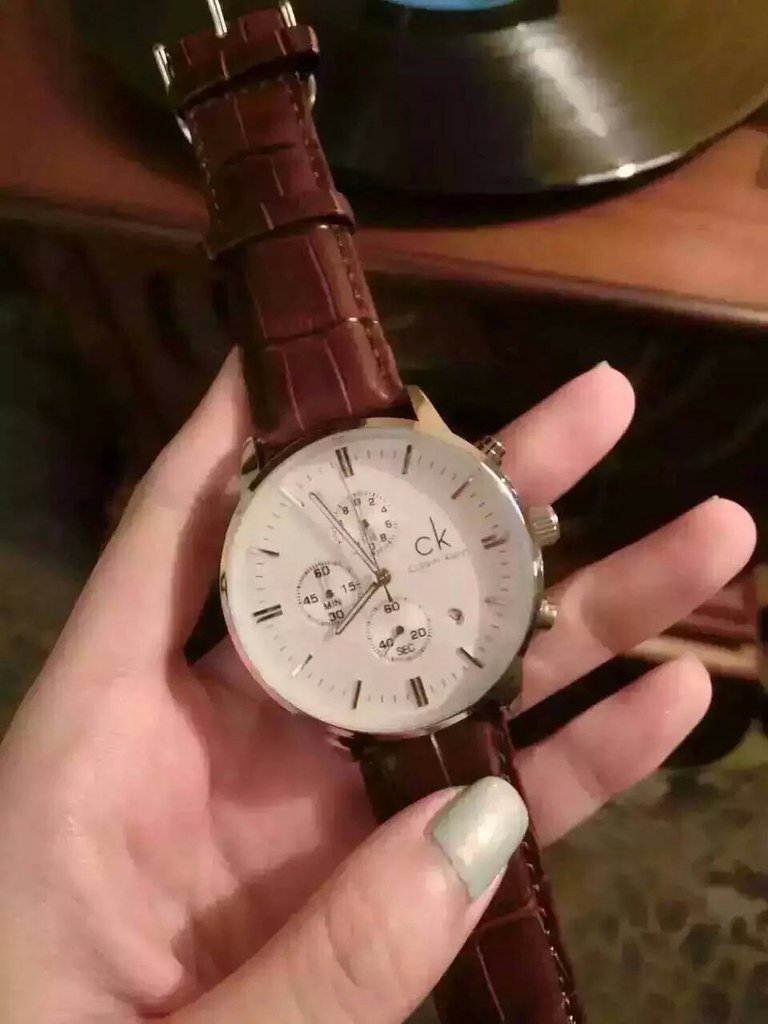A woman is holding a Calvin Klein watch in her left hand, with her thumb resting on top of the watch face and her fingers supporting it from the back. Her thumb is adorned with a long, moss green nail, while her other nails appear to be shorter and unpainted. The watch band is made of brown leather, and its circular white face is notably large. 

The watch face features alternating single and double lines to mark the hours, with double lines at 12 o'clock and 3 o'clock, and single lines at 1 o'clock and 2 o'clock, creating a distinctive pattern around the dial. Some of these hour markers are beginning to fade, suggesting that the watch is older. 

Three small sub-dials are embedded within the watch face. The bottom sub-dial tracks the seconds, while the right one counts minutes in increments of 15, with markings at 15, 30, 45, and 60. The top sub-dial displays hours in a 24-hour format, marked with even numbers from 2 to 12. It indicates the current time as approximately 6:55. 

In the background, an entertainment center or table is visible, with a silver object placed on it. The floor beneath the table is covered with a floral patterned rug.